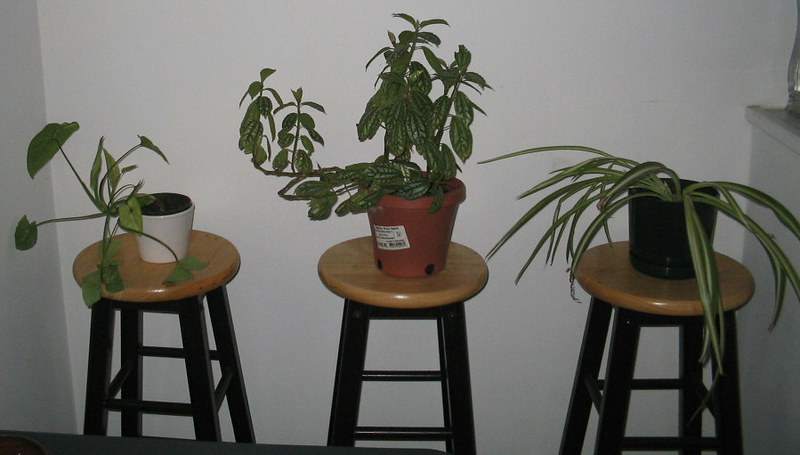The image depicts an indoor scene with a white wall in the background. Three wooden stools with black legs and round oak-finished seats are positioned in the center of the frame. Each stool supports a distinct potted plant. The stool on the left features a small white pot containing a green plant with long stems and leaves. The middle stool holds a larger reddish clay pot—potentially plastic mimicking clay—home to a plant with what appear to be basil leaves. Lastly, the stool on the right has a black pot, possibly plastic, with a plant resembling a snake plant, its long green leaves with white centers cascading over the stool's edge. A gray counter or cabinet is partially visible on the right, connecting to the wall.